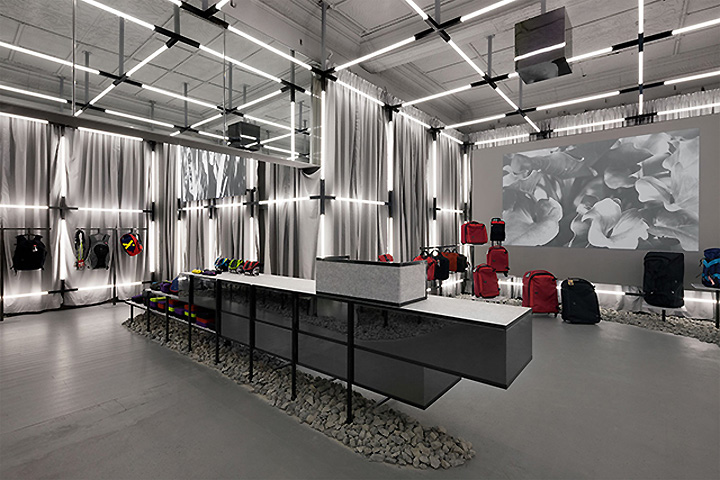The image depicts an industrial-themed showroom with predominantly gray tones throughout the space. The large, open room has all its windows covered with gray curtains, and the floor is uniformly tiled in gray. Ceiling lights, which are cylindrical and alternate between black and white at their joints, crisscross overhead, casting a soft industrial glow on the room.

On the left side of the image, numerous suitcases are displayed, featuring black and red colors. Alongside these are some racks with a variety of backpacks in black, gray, and red. There is also mention of folded clothing and various accessories on the left side, hinting at a multi-purpose display setup for small items.

In the center of the room sits a rectangular display structure that houses a collection of objects in red, turquoise, green, and purple. This structure is situated on a narrow strip of gray rocks embedded into the floor, adding to the room's industrial aesthetic. Some shelving units are placed on top of this rocky base, possibly showcasing the colorful objects more prominently.

The right side of the room features a large screen or possibly a poster with a black and white floral design, mounted on a gray wall. Below this display area is a meticulously arranged layout of red and black luggage, further emphasizing the showroom’s focus on travel accessories.

In summary, the image captures a meticulously arranged, industrial-style showroom predominantly in gray, punctuated with colorful travel gear and accessories, illuminated by a unique ceiling light arrangement.